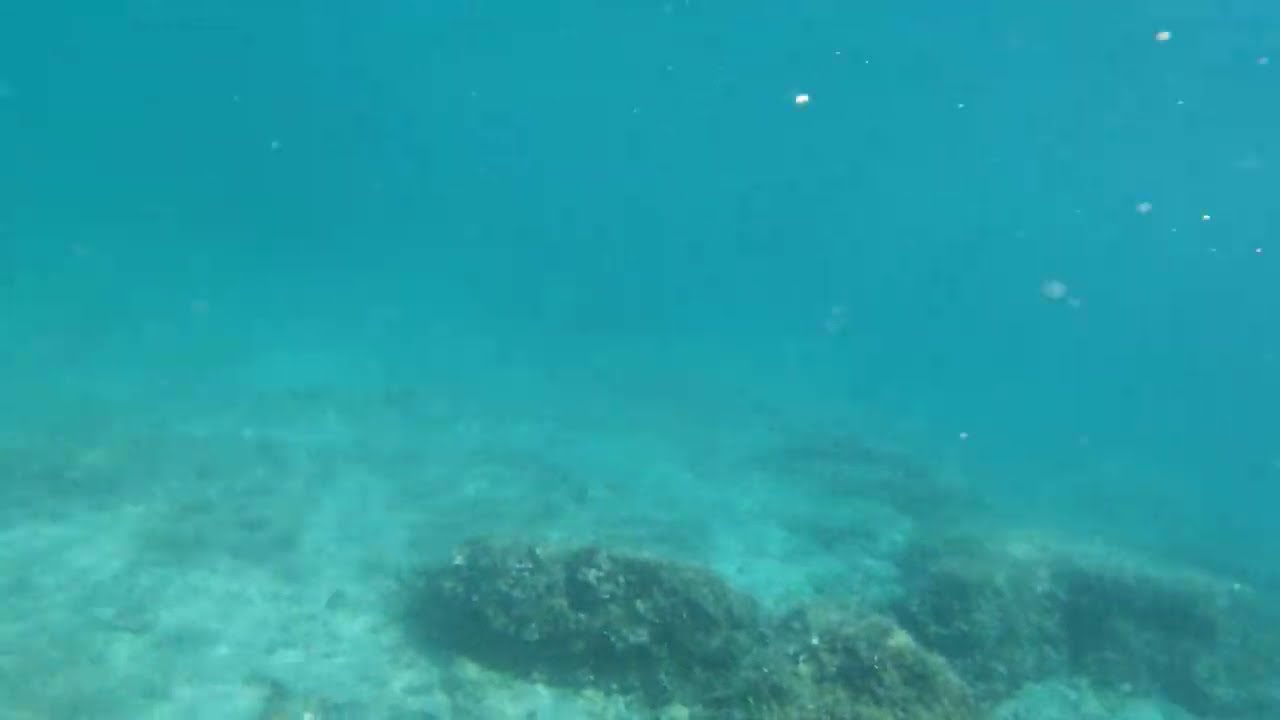This image captures an underwater scene with a somewhat clear yet murky quality. The upper half of the image is dominated by a deep blue or teal color, transitioning to a lighter shade as it moves towards the seafloor. This seafloor appears rocky, interspersed with patches of dark green moss or mildew and areas of dark brown and sandy white, though the sand is tinted blue from the water above. Scattered throughout the water are tiny white bubbles, reminiscent of stars in the night sky, mainly concentrated in the upper corners of the image. The background is blurred, limiting the visibility to the foreground and a small portion of the mid-ground, reinforcing the sense of underwater depth.